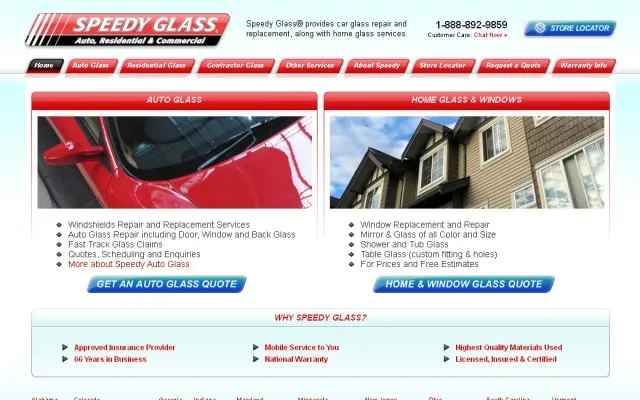This is a detailed description of a website for a company specializing in glass repair and replacement services. 

The header section features a pale glass-blue background with a green base, transitioning into a red background encircled by a black border. The bottom portion of the header showcases "Speedy Glass" in white text, underneath which the services offered are listed: auto, residential, and commercial. Surrounding this, a message reads, "Speedy Glass provides car glass repair and replacement along with home glass services." The contact number, 1-888-892-9859, is prominently displayed alongside a red "Chat Now" button.

Further down, a blue banner with white text reads "Store Locator." Below this, a navigation menu includes links to Home, Auto Glass, Residential Glass, Contractor Glass, Other Services, About Speedy, Store Locator, Request a Quote, and Warranty Info.

The main banner highlights "Auto Glass" and features an image of a car, followed by five bullet points elaborating on the services: More About Safety, Auto Glass Quotes and Scheduling, Inquiries, Fast Track Glass Claims, Auto Glass Repair, Windshield Repair and Replacement Services. Additionally, information about "Window Replacement" is shown, detailing services for home glass windows, table glass, custom fittings and holes, prices and fees estimates, shower and tub glass, mirror glass of all colors and sizes, window replacement, repair, and home window glass flip.